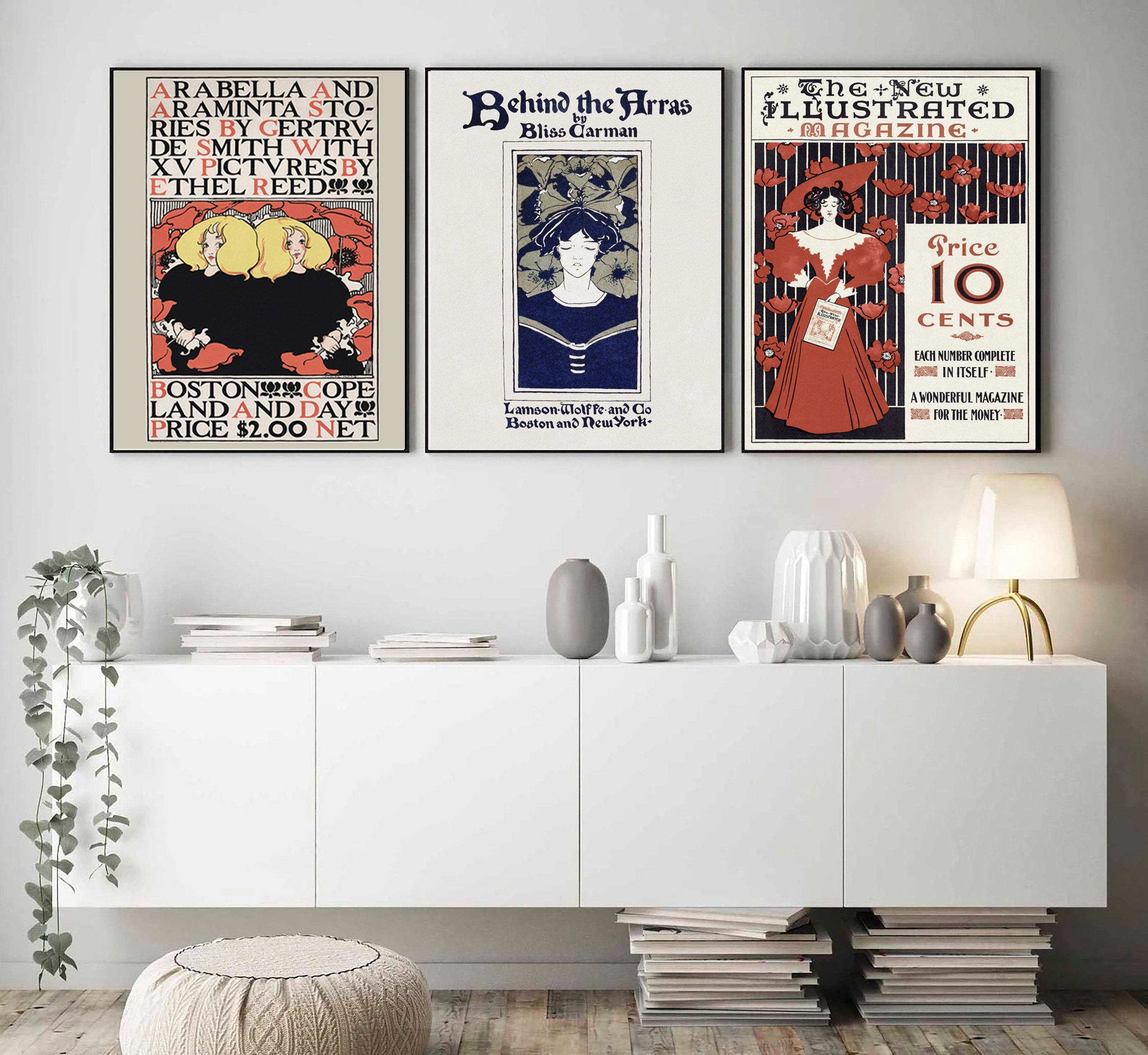The image showcases a meticulously arranged indoor setting, likely styled by an interior decorator. The focal point is a pristine white wall adorned with three framed portraits hung in a row. Each black-framed portrait features illustrations of women and distinctive text. The leftmost portrait depicts a cartoon of two women with blonde hair and the text "Arabella and Araminta Stories by Gentry D. Smith" accompanied by "15 Pictures by Ethel Reed." The central portrait bears a white background with a person in blue amidst flowers, titled "Behind the Eras by Bliss Carmen." The rightmost portrait showcases a woman in a red dress with the title "The New Illustrated Magazine" and a price of 10 cents.

Directly beneath the portraits is a sleek, white, floating shelving unit. This unit, composed of white squares, holds various decorative items: a lamp, a mix of gray and white vases, a stack of books, and a white planter housing a lush green plant with trailing vines. A beige ottoman sits on the weathered, light-colored wooden floor, drawing attention to its cozy yet stylish addition to the scene. Underneath the shelving unit, two neat stacks of books are visible, further enhancing the room's curated aesthetic.